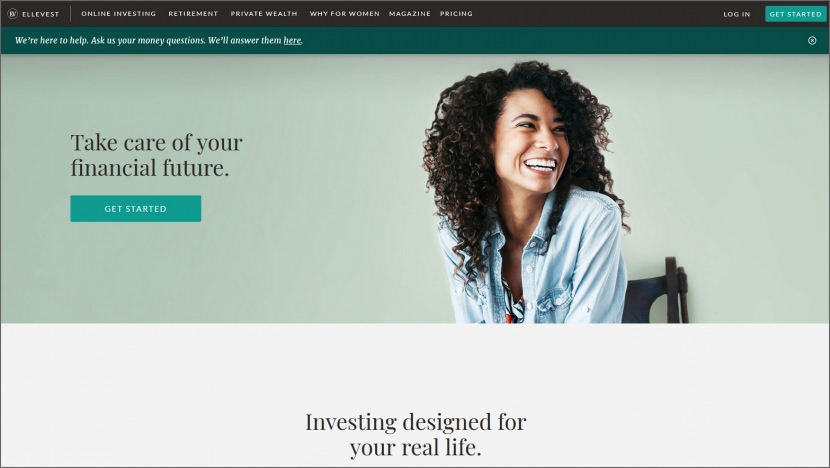The website, designed to help manage finances, features an inviting layout centered around a clean and modern aesthetic. Dominating the right-hand side of the page is a vibrant photo of a young, smiling woman with long, dark, curly hair. Her broad, open-mouthed smile showcases straight white teeth, and she appears to be glancing at someone off-screen over her left shoulder. Dressed in a light blue, chambray-style button-up shirt and sitting in a black chair, she exudes a welcoming and approachable demeanor. The background behind her is minimally visible, maintaining focus on her cheerful expression.

The website’s color scheme includes a light green area where the woman is placed, enhancing the tranquil and friendly atmosphere. A prominent feature is a broad white bar at the bottom center, displaying the tagline: "Investing designed for your real life."

To the left of the woman’s image, a set of impactful lettering stands out, reading: "Take care of your financial future," accompanied by a conspicuous "Get Started" button beneath it. Above, a darker green banner stretches across the top of the page, boldly stating: "We're here to help. Ask us your money questions," with an inviting link to provide answers.

In the top right corner, users can easily find options like "Login" and "Get Started" links. The website's navigation is streamlined at the top with various tabs including "Online Investing," "Retirement," "Private Wealth," "Wise Women," "Magazine," and "Pricing."

In the top left, the company's name, "Ellevest," is prominently displayed, suggesting this is the financial investment firm’s official website. The overall design is user-friendly, aiming to empower users to manage their financial future confidently.